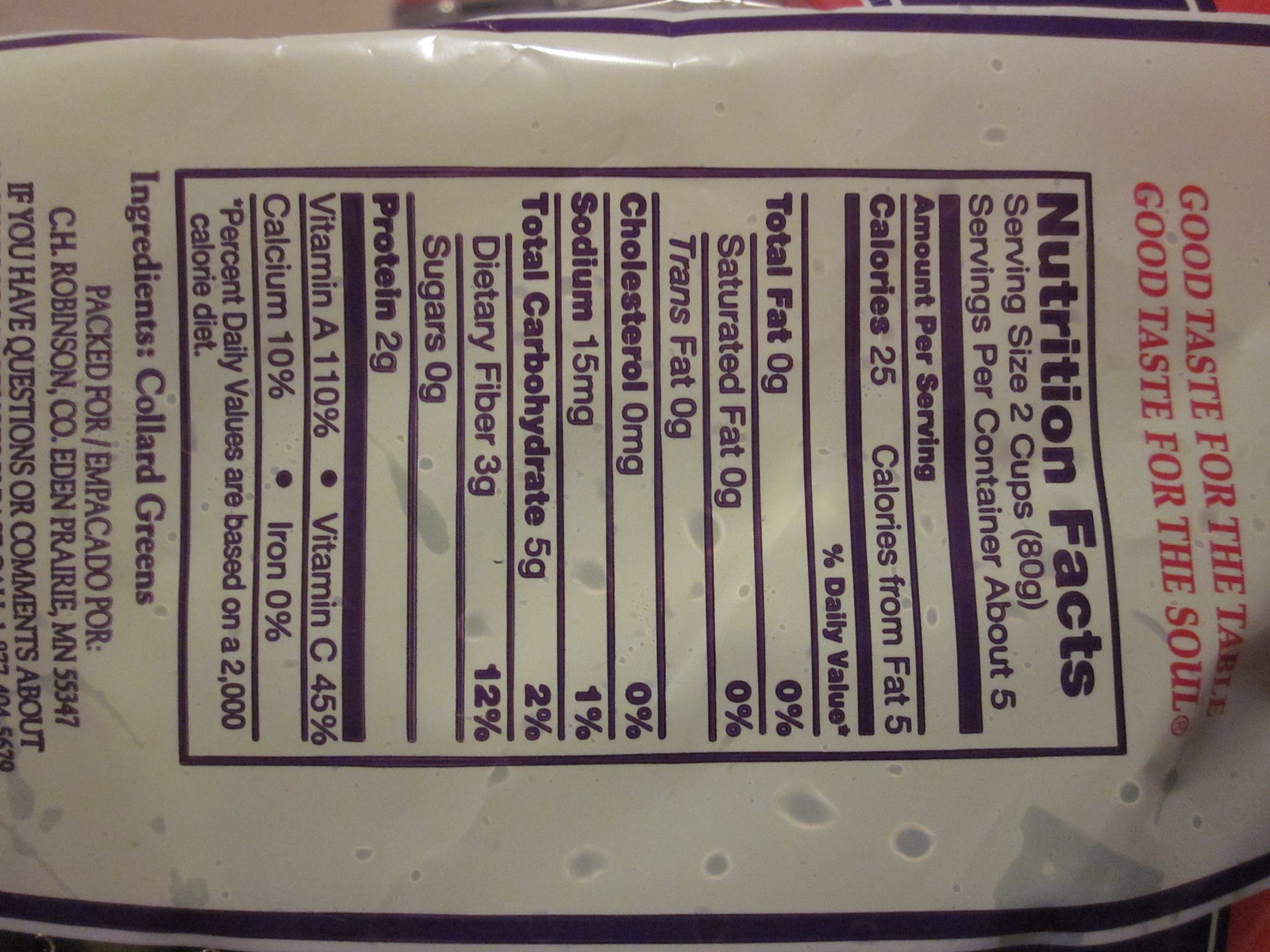This is a detailed photograph of a sideways bag of collard greens. At the top of the bag, in red letters, it reads, "Good Taste for the Table, Good Taste for the Soul." The bag features a blue border on its sides and is packed for Empicado Poor by C.H. Robinson Company, located in Eden Prairie, Minnesota, 55347. 

Visible through the white plastic, you can see water droplets on the collard greens. The central focus of the image is a Nutrition Facts label with black text and large bold blue letters. The label details that a serving size is 80 grams, which provides 25 calories, including 5 calories from fat. It includes the following nutritional information: total fat 0 grams, 0% (saturated fat 0 grams, 0%; trans fat 0 grams), cholesterol 0 milligrams, sodium 15 milligrams, total carbohydrates 5 grams, 2% (dietary fiber 3 grams, 12%; sugars 0 grams), and protein 2 grams. It also lists vitamin A at 102%, vitamin C at 45%, calcium at 10%, and iron at 0%. The label concludes with a note that the percent daily values are based on a 2,000 calorie diet.